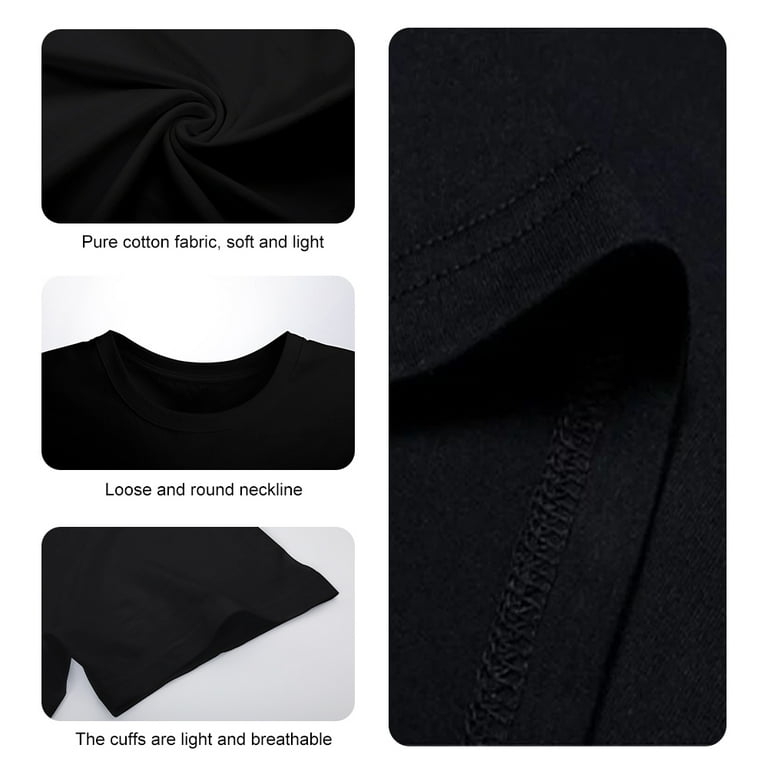This is a product advertisement image showcasing the features of a black t-shirt against a white background. The layout comprises four images: three smaller rectangular pictures aligned vertically on the left and one longer rectangular picture on the right.

- The top-left image depicts the black t-shirt twisted into a knot to emphasize its texture, with the caption "Pure cotton fabric, soft and light" in black text.
- The middle-left image focuses on the neck area, highlighting a "loose and round neckline" as described underneath.
- The bottom-left image captures the hem of the t-shirt, specifically the cuffs, with a label stating "the cuffs are light and breathable."
- On the right, a single elongated image provides a close-up of the t-shirt's stitching, showcasing the craftsmanship and durability of the seams.

The overall presentation effectively displays the t-shirt's quality and comfort through detailed and zoomed-in views of its fabric, neckline, cuffs, and stitching.